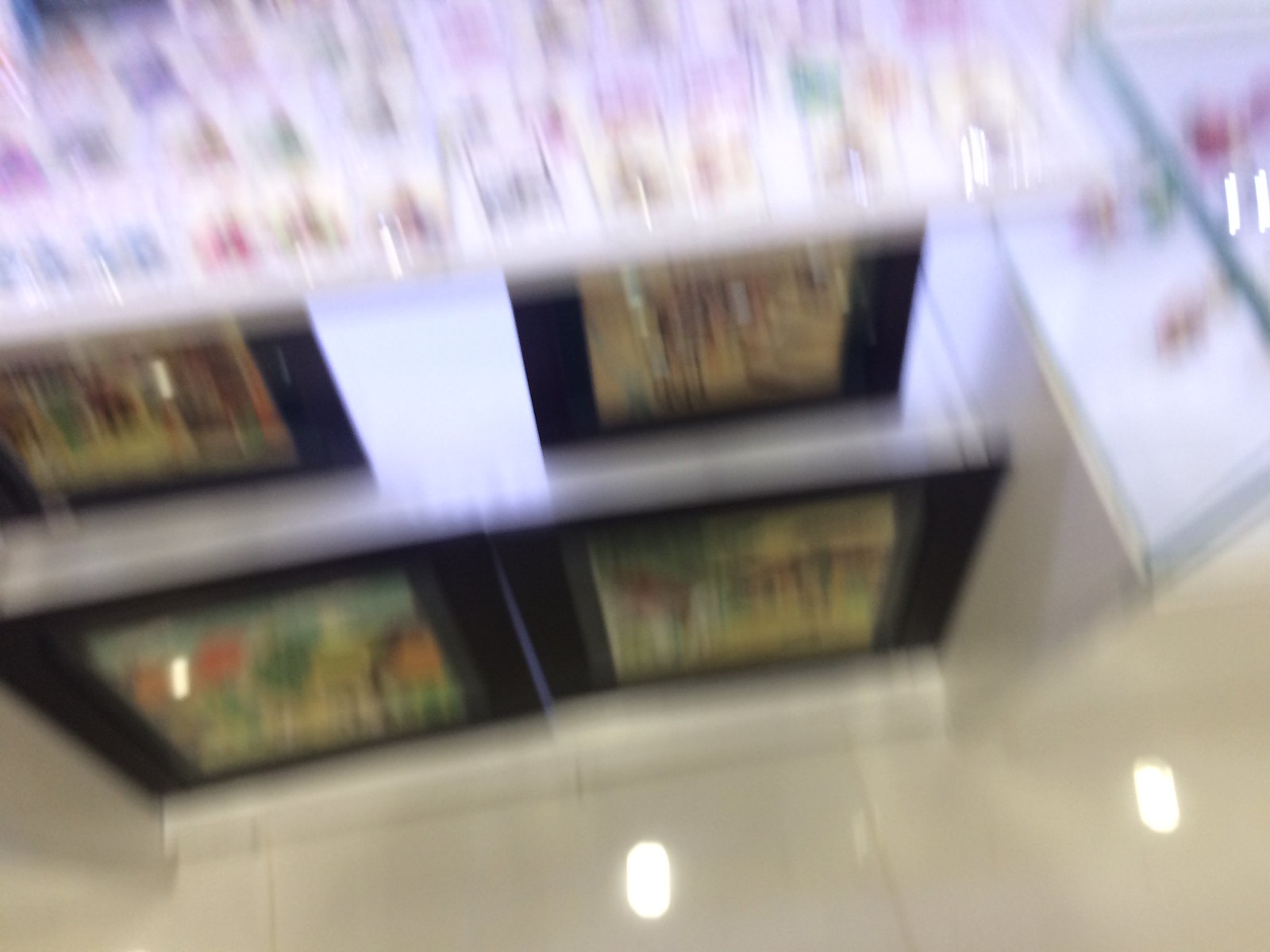This image is a blurry top-down view of a shop display set up in a brightly lit area. The photo has a rectangular shape with the top and bottom sides longer than the left and right sides. The bottom portion of the image clearly showcases glossy square-shaped white tiles reflecting the overhead lighting in circular patterns. Towards the top half of the image, a rectangular white pedestal with a see-through glass case is visible in the top right corner, containing various indistinguishable objects due to the blurriness of the photo.

At the forefront of the image, there is a multi-tiered table. On the top tier, there are a couple of boxes with a smaller table positioned atop them. This smaller table holds several small bottles, which might be nail polish or perfume, presenting a mix of different colors—reds, greens, and yellows. The lower tier, as well as the floor beneath it, holds four items that resemble framed drawings or pictures, surrounded by thick black frames. The drawings feature colors like greens, oranges, and browns, although the overall blur makes detailed identification challenging. The scene indicates a busy, well-lit store or department area with diverse product displays and vibrant lighting.